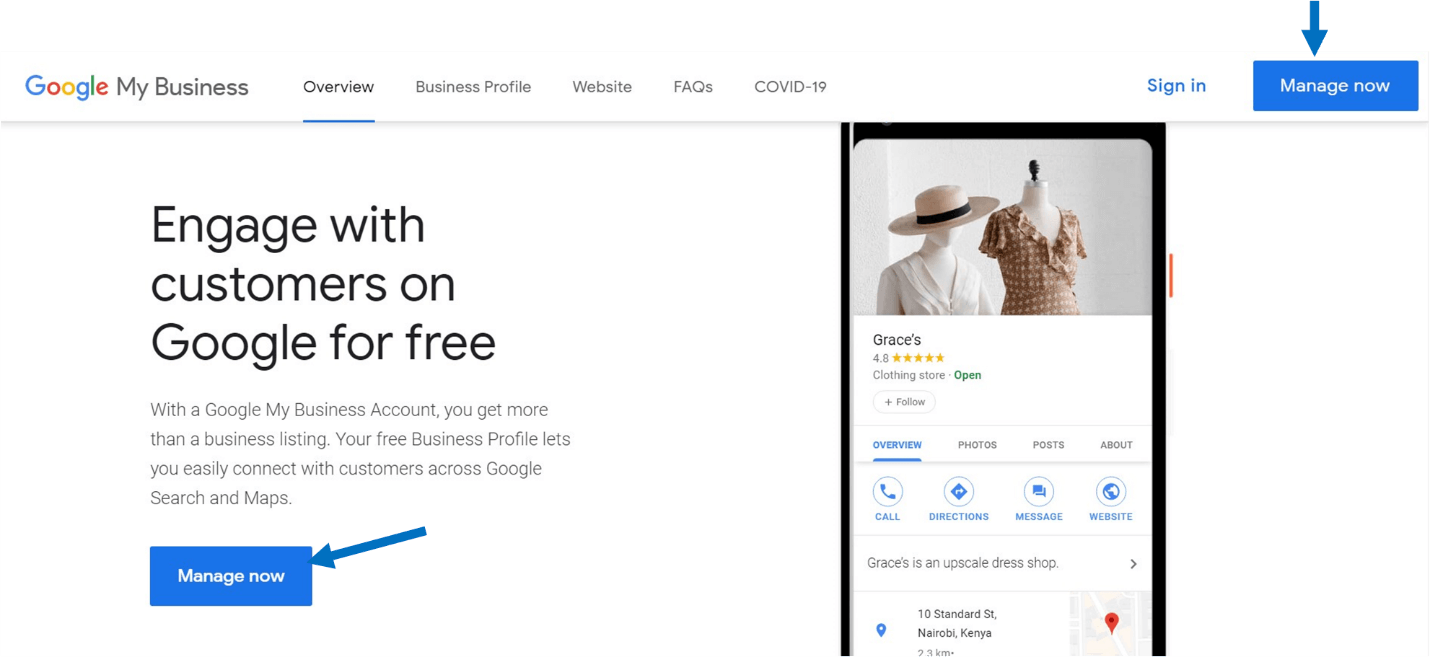This screenshot showcases the Google My Business website interface. At the top of the page, there's a toolbar featuring the Google logo on the left, followed by the words "Google My Business." The toolbar also includes menu options such as Overview, Business Profile, Website, FAQs, and COVID-19. On the right side, there's a Sign-In link and a prominent blue "Manage Now" button, indicated by a blue arrow.

The main section of the page highlights the Overview tab, which is currently selected. On the left side, a header reads, "Engage with customers on Google for free." Below that, a statement explains the benefits of a Google My Business account, emphasizing the ability to connect with customers across Google Search and Maps, all free of charge. Another blue "Manage Now" button is visible, also marked with a blue arrow for emphasis.

On the right side of the screenshot, there’s an image of a smartphone display. The phone screen shows a business listing for "Gracie," a clothing store rated 4.8 stars, marked as open, with a "Follow" button. The options Overview (highlighted), Photos, Posts, and About are displayed beneath the store name. The Overview section provides quick access options like calling, getting directions, messaging, or visiting the website. The description underneath reads, "Gracie's is an upscale dress shop," with a forward arrow hinting at additional details. The listing also includes the store's address and a small map thumbnail with a location pin.